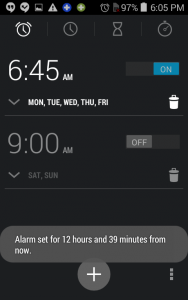The screen displayed on the cell phone showcases a standard interface packed with various icons and information, essential for seamless usability. At the top of the screen, a row of icons provides quick access to different functionalities: a speech bubble icon for messaging, a graph icon perhaps for analytics or reports, a triangle icon whose purpose remains unspecified, a plus sign possibly indicating help or additional features, and a green circular button that likely represents the phone's status. To the right of the screen, typical cell phone information is displayed, including the current time, 6:05 PM, the battery percentage at 97%, and a battery life symbol.

Just below these elements, there is a second row featuring four intuitive icons for time management: an alarm clock, a basic clock, an hourglass for setting timers or countdowns, and a stopwatch symbol designated for timing events. 

Below this row, the screen shows a detailed schedule of alarms. The first alarm is set for 6:45 AM and is activated, indicated by an 'On' button, with notifications scheduled for weekdays, Monday through Friday. Adjacent to this entry is a trash can icon, a clear option for deleting the alarm. The next alarm is set for 9:00 AM but is turned off, as indicated by the grayed-out button, and is configured for weekends, Saturday and Sunday, with its own deletion option.

Further down, there is a note highlighting an alarm scheduled to trigger in 12 hours and 35 minutes from the current time, aligning correctly with the 6:05 PM timestamp given that it's set for 6:45 AM the next day. At the bottom of the screen, a plus sign encourages the addition of new alarms, and three vertically aligned dots provide access to broader options and settings.